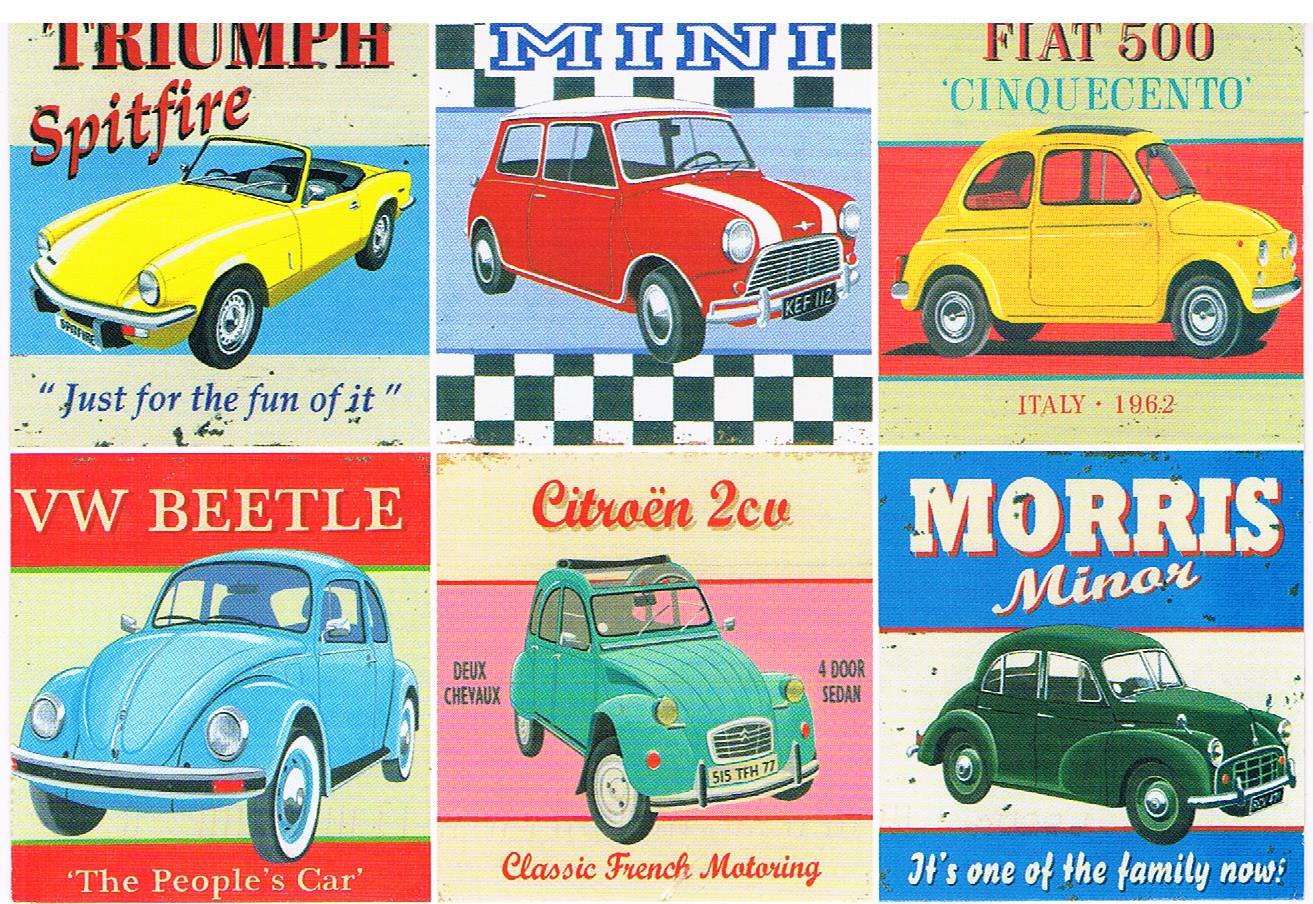This image is a six-frame collection of vintage automobile illustrations, arranged in two rows of three. In the top left frame, there's a yellow Triumph Spitfire, a two-seater convertible with the phrase "Just for the fun of it" underneath. Adjacent to it, on the right, is a red Mini Cooper featuring black and white checkerboard stripes and blue lettering on its sign. The frame next to the Mini displays a yellow Fiat 500, labeled "Cinquecento" and "Italy 1962," capturing the classic design of this iconic car.

The bottom row starts with a light blue Volkswagen Beetle on the left, accompanied by the caption "The People's Car." Next to it, in the middle frame, is a Citroen 2CV, a four-door sedan with a cloth sunroof, presented as "Classic French Motoring" with some French text. Finally, the bottom right frame features a Morris Minor, a green car with the caption "It's one of the family now," completing this nostalgic showcase of European automotive classics.